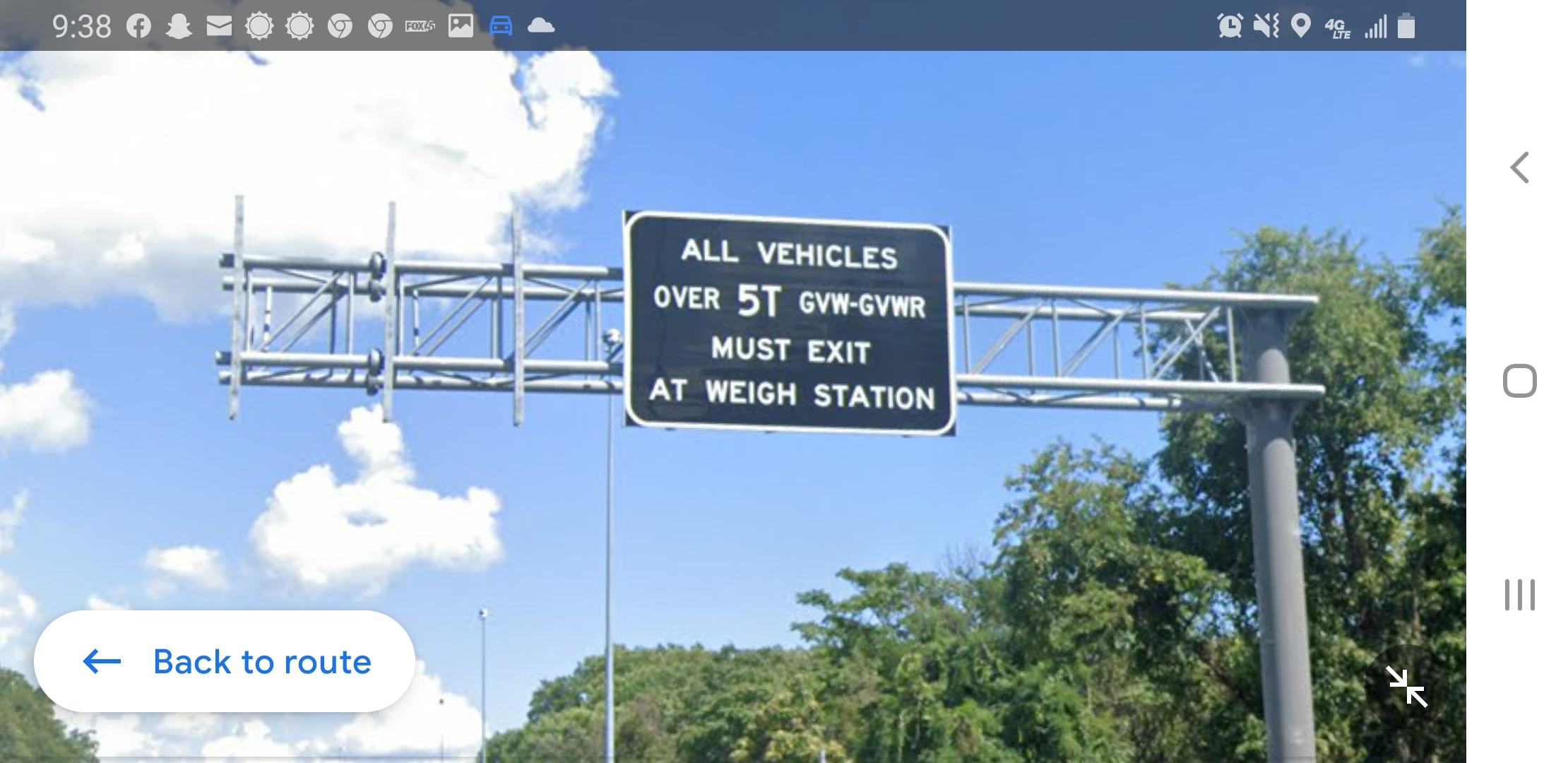This is a color, horizontal screenshot of a mobile device display, taken at 9:38 AM. The top bar showcases an array of icons, including Facebook, Snapchat, email, weather with two sun symbols, Google Chrome, battery life, signal strength, 4G LTE connectivity, a map icon, a sound icon, and a clock. The main content of the screenshot centers on a photograph of a black street sign with white block letters mounted on a large metal pole. The sign reads, "All vehicles over 5 tons, GVW-GVWR, must exit at Weigh Station," with two arrows pointing towards each other. In the lower right-hand corner, there's a circular symbol, while the lower left-hand corner features a white pill-shaped button with blue text that reads, "Back to Route," accompanied by a left-pointing arrow. The background displays a clear blue sky with a scattering of white clouds and trees extending from the right corner to the center of the image. Additional interface elements include a square, a hamburger menu, and a left-pointing arrow in light gray on a white background.